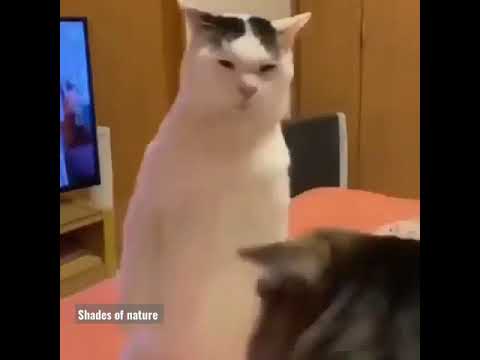The image is a somewhat fuzzy and out-of-focus shot featuring two cats in what appears to be a room. The main focus is on a white cat with black spots on either side of its head, standing on its back legs on a pink surface, which might be a table or the edge of a bed. The cat appears unhappy, its dark eyes squinting and ears positioned downwards, giving an angry expression. To the bottom right of the frame, we see only the flat ear and the top of the head of a second cat, which has dark fur and seems to be facing away from the camera. The background includes a black chair behind the white cat on the right, and a cropped TV set with a show on the left, sitting on a TV console. The wall behind them is paneled with brown, possibly wooden, boards. The image is bordered by thick black bars on the right and left sides, and features the text "shades of nature" in white with a semi-transparent black background in the lower left-hand corner.